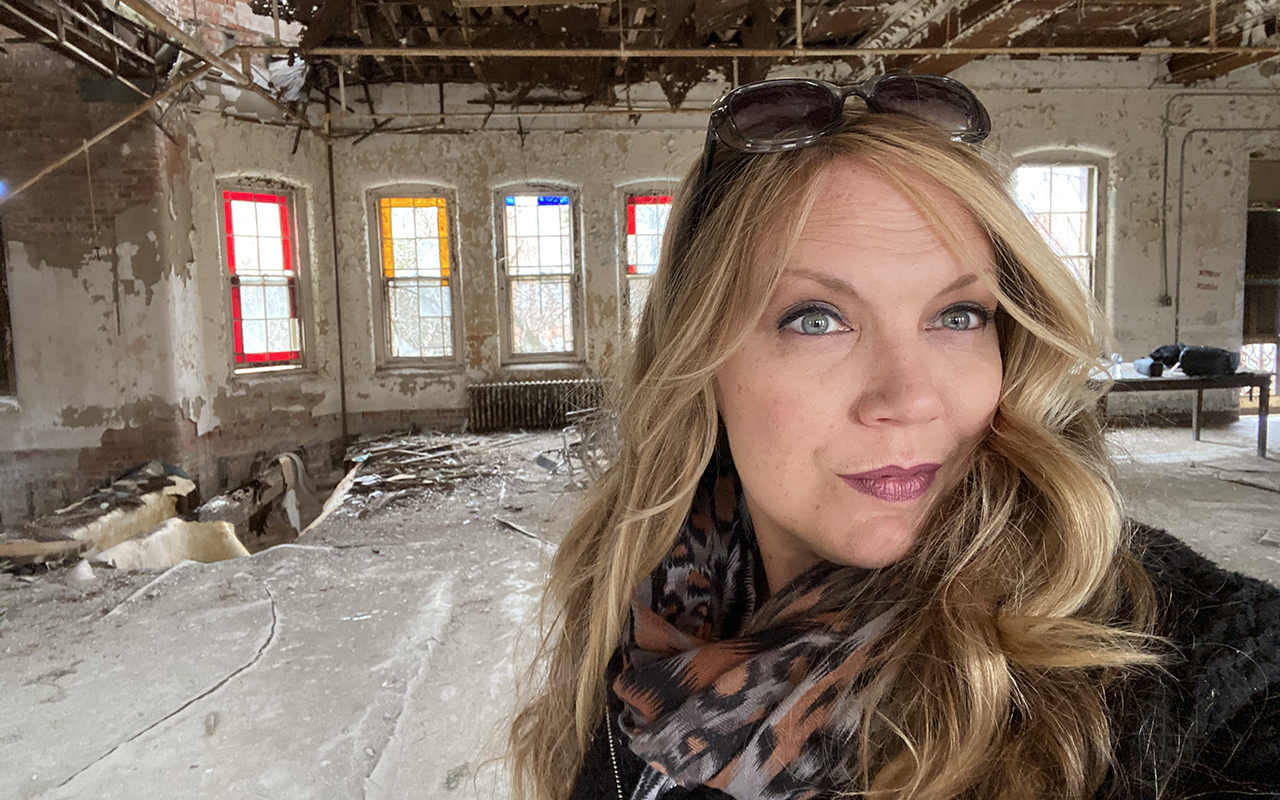The image is a horizontally aligned rectangular close-up of a woman likely taking a selfie in a room under construction. She is positioned to the right-hand side. The background features a series of six vertical rectangular stained-glass windows with various colors, including red, yellow, and blue frames. The ceiling is stripped down to exposed bars, and the floor appears to be cracked cement or concrete with a visible dip under the windows, suggesting ongoing ground work. The room also has a table on the right-hand side.

The woman, who appears to be in her 40s, has long, curly or wavy blonde hair and bluish-green eyes. She is smiling slightly at the camera. Sunglasses rest on top of her head, and she wears a cheetah-patterned scarf around her neck along with what seems to be a black coat, although her body is mostly out of frame.